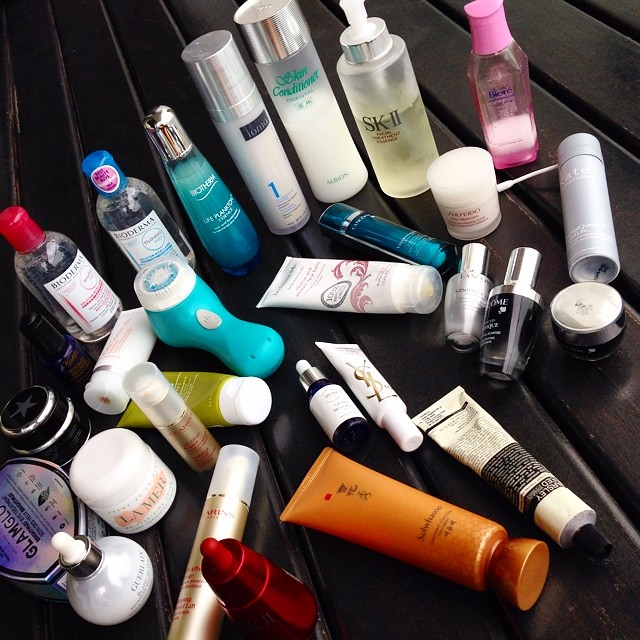The image features a meticulously arranged collection of beauty products displayed on a sleek, black wooden table composed of joined planks, creating a sophisticated backdrop. In the back row, an assortment of bottles is thoughtfully positioned upright. These include both squeeze bottles and elegant glass pump bottles, each adorned with lids. The bottles stand out in various colors: some are white with green lettering, others are a vibrant turquoise, and a few exhibit a charming combination of pink and white labels.

In front of these upright bottles, several squeeze bottles are laid flat on the table. The color palette here is equally diverse, featuring metallic gold alongside elegant pink and white designs. Among these is a selection of small tubes, including a notable lip tube from Yves Saint Laurent, distinguished by its luxurious white and gold lettering.

Positioned to the left are several jars with screw lids, adding further variety to the display. These containers predominantly feature white with pink and gold accents, completing this visually appealing and orderly presentation of beauty products.